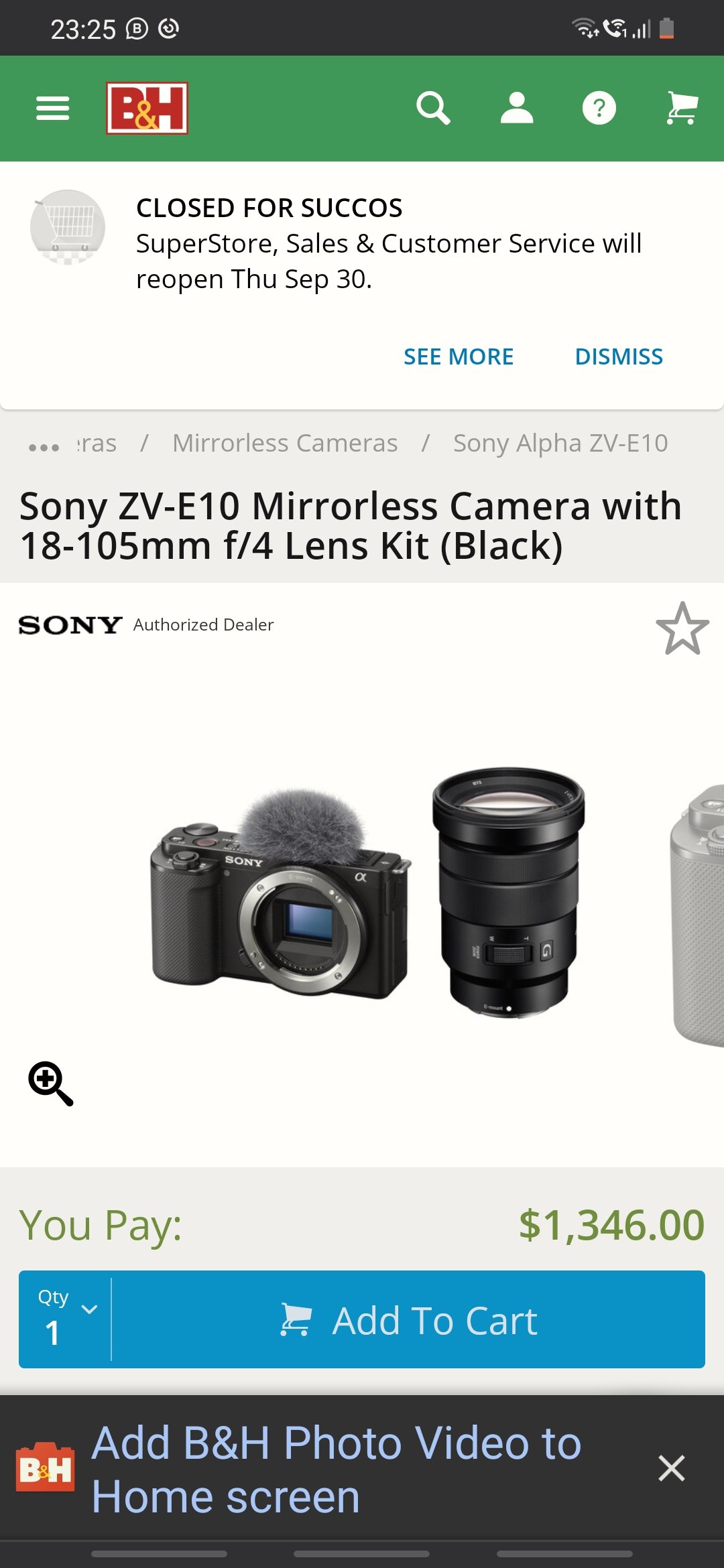The screenshot displays a webpage listing for a Sony ZV-E10 mirrorless camera with an 18-105mm f/4 lens kit in black. The listing, accessed on a smartphone, features various interface elements from the B&H Electronics website. At the top, there is a notification that reads, "Closed for Sucos, superstore sales and customer service will reopen Thursday, September 30th." The screen shows the time as 23:25, with indicators for barcode scanning, battery life, a shopping cart, and a search function. 

The core of the image prominently centers on the camera and lens kit. Pricing information is clearly presented in a gray banner with green text stating, "You pay $1,346." Below this, within a blue rectangle, options for "Quantity: 1" and an "Add to Cart" button accompanied by a shopping cart icon are visible. Towards the bottom of the screen, another gray banner features bluish text suggesting, "Add B&H Photo Video to home screen," with a white 'X' symbol on the right for dismissal. An enlarge button, "See More," and dismiss options are also part of the interface. The distinctive red B&H logo appears both at the top and bottom of this detailed product listing.